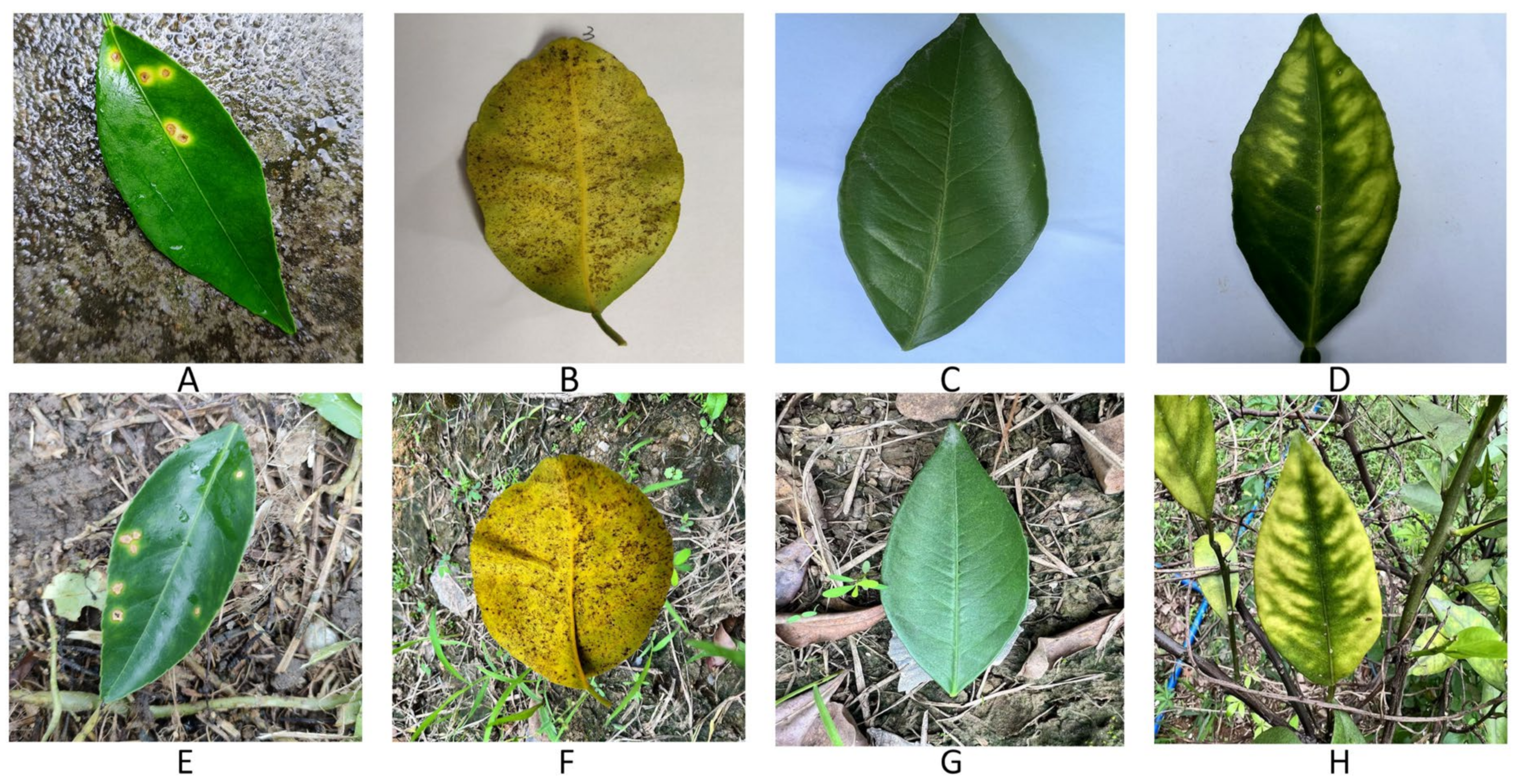The image is a detailed collage of eight distinct leaves, arranged in two horizontal rows with four leaves each, delineated by white lines. Each leaf is labeled sequentially from A to H. The top row (A, B, C, D) showcases leaves that have been plucked, while the bottom row (E, F, G, H) displays leaves still growing on their respective plants. 

Leaf A is an oval-shaped green leaf with yellow and red spots, set against a backdrop of a grayish, mossy rock. Leaf B is more rounded and exhibits a yellow hue with brown spots. Leaf C represents a typical green leaf, whereas Leaf D is a slightly shiny, curled green leaf with yellow accents. The bottom row mirrors the top row, but the leaves appear more vibrant and alive. Leaf E mirrors A with its spotted appearance. Leaf F resembles B with its yellow and brown coloration. Leaf G looks much like C, showcasing a simple green leaf, while Leaf H, like D, is a green leaf with yellow accents, appearing shinier and slightly curled. The juxtaposition highlights the contrast between the plucked leaves and those still thriving on their plants.